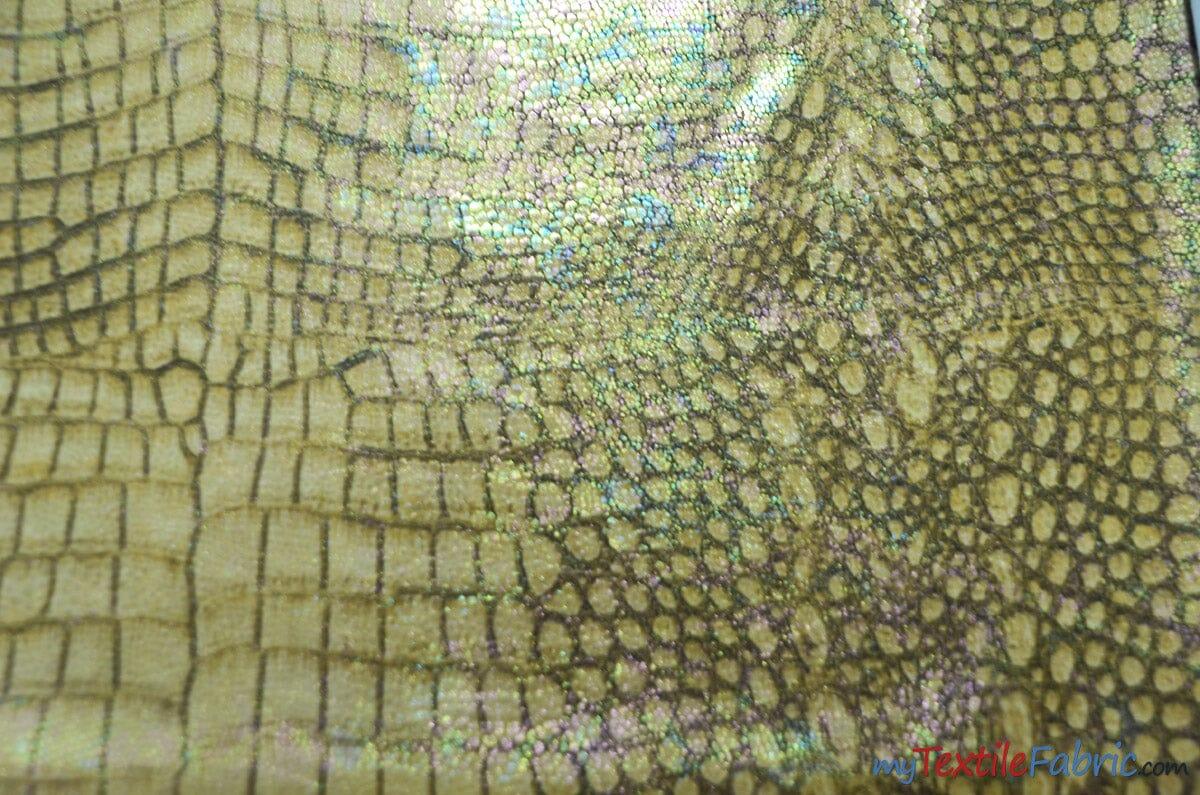This photograph captures a close-up of a fabric designed to imitate reptile skin, possibly alligator or snake skin. The horizontally aligned rectangular image features a detailed scaly pattern with varying colors: light brown cells bordered by darker greenish-brown hues. The scales, with a mix of square and circular patterns, display a striking rainbow-like, iridescent reflection, particularly prominent in the top center section and slightly down the center and right-hand side. Shimmering beads in shades of white, blue, and light purple are also visible towards the top center of the fabric, adding a glittery effect. In the lower right corner, a watermark reads "mytextilefabric.com" with 'my' in blue, 'textile' in red, 'fabric' in blue, and 'dot-com' in black, standing out against the busy background. The fabric's overall design combines a mix of textures and colors, making it challenging to discern if it's a genuine reptile skin or an expertly crafted textile.